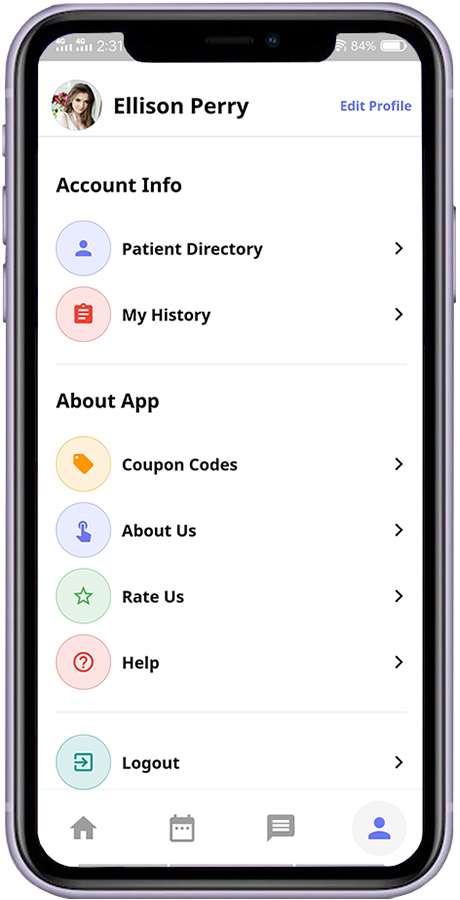The image captures a user profile interface for Allison Perry within a mobile application. At the top of the screen, the status bar displays the time (2:31), 4G Wi-Fi connectivity, and a battery life indicator showing 84%.

In the center of the screen, Allison Perry's profile picture is positioned to the left, next to her name displayed prominently. To the right is an "Edit Profile" button. Below this, several sections of account information are neatly arranged: "Patient Directory" and "My History," both in bold black text. To the left of "Patient Directory" is a generic blue avatar icon, while "My History" is marked by a red clipboard icon. Each section has right arrows indicating further details can be accessed.

A faint dividing line separates these sections from the "About App" area, which includes multiple functionalities: a coupon icon accompanied by "Coupon Code," an icon of a finger pressing a button labeled "About Us," a star icon for "Rate Us," and a logout option. Below is a navigation bar with icons for Home, Calendar, Text Messaging, and User Information, with the latter highlighted in blue indicating the current section.

The overall background is white, except for the colored icons to the left of each label: blue for user-related sections, red for history, and grey for utility options like logout and help.